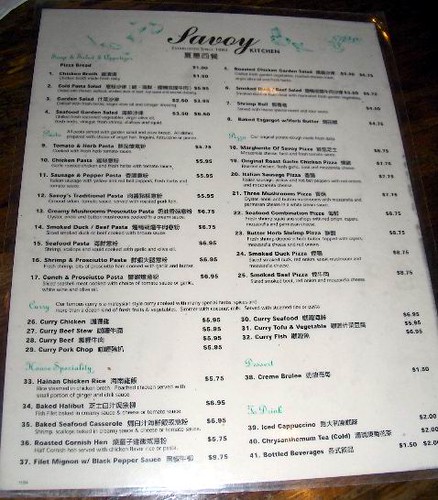The image features a menu from Lavoie Kitchens, presenting an assortment of dishes with descriptions in both English and Chinese. The menu is predominantly white with black text, accented by green elements that serve to delineate sections such as "Specialty" and possibly other categories. The menu is placed on a wooden table surface.

The photograph of the menu appears on the viewer's screen with approximate dimensions of 3 inches horizontally and over 4 inches vertically. The detailed offerings include dishes like curry seafood, curry beef, and a three mushroom pizza. Notably, one of the highlighted items is filet mignon with black pepper sauce, priced at just $9.75. While the prices seem quite reasonable, they may indicate smaller serving sizes, or the menu could potentially be from an earlier time, as there is no date provided for context.